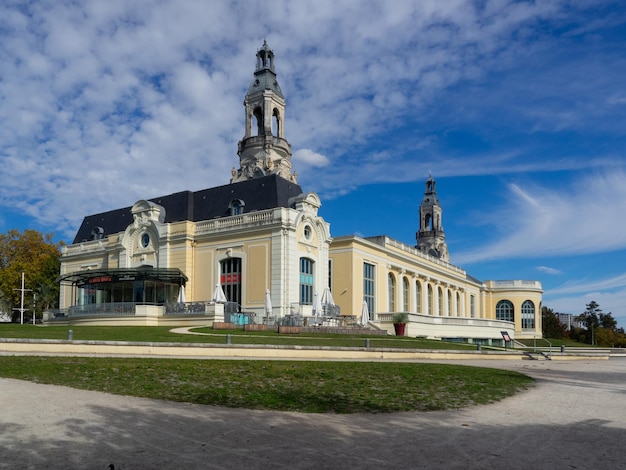In this vibrant real-life image, we see an elegant vintage church-style building, potentially from the early 1920s, characterized by its distinct yellow and white paint. This architectural gem boasts two prominent chapel pillars or bell towers, and its design is resonant of early 20th-century architecture. 

The church has three stories with large arched windows, including an oval-shaped extension with stained glass windows on the right center. The structure displays a lattice railing at the very top of its front, just above the semi-circular archway that extends over the sidewalk. The building’s black roof tops it off with an air of historic grandeur.

In the forefront, there is a driveway bordered by a meticulously kept lawn, leading to a patch of grass and a fence, framed by trees on both sides. The scene is set against a backdrop of a vibrant blue sky with scattered clouds, providing a picturesque and serene atmosphere to this beautifully maintained architectural relic.